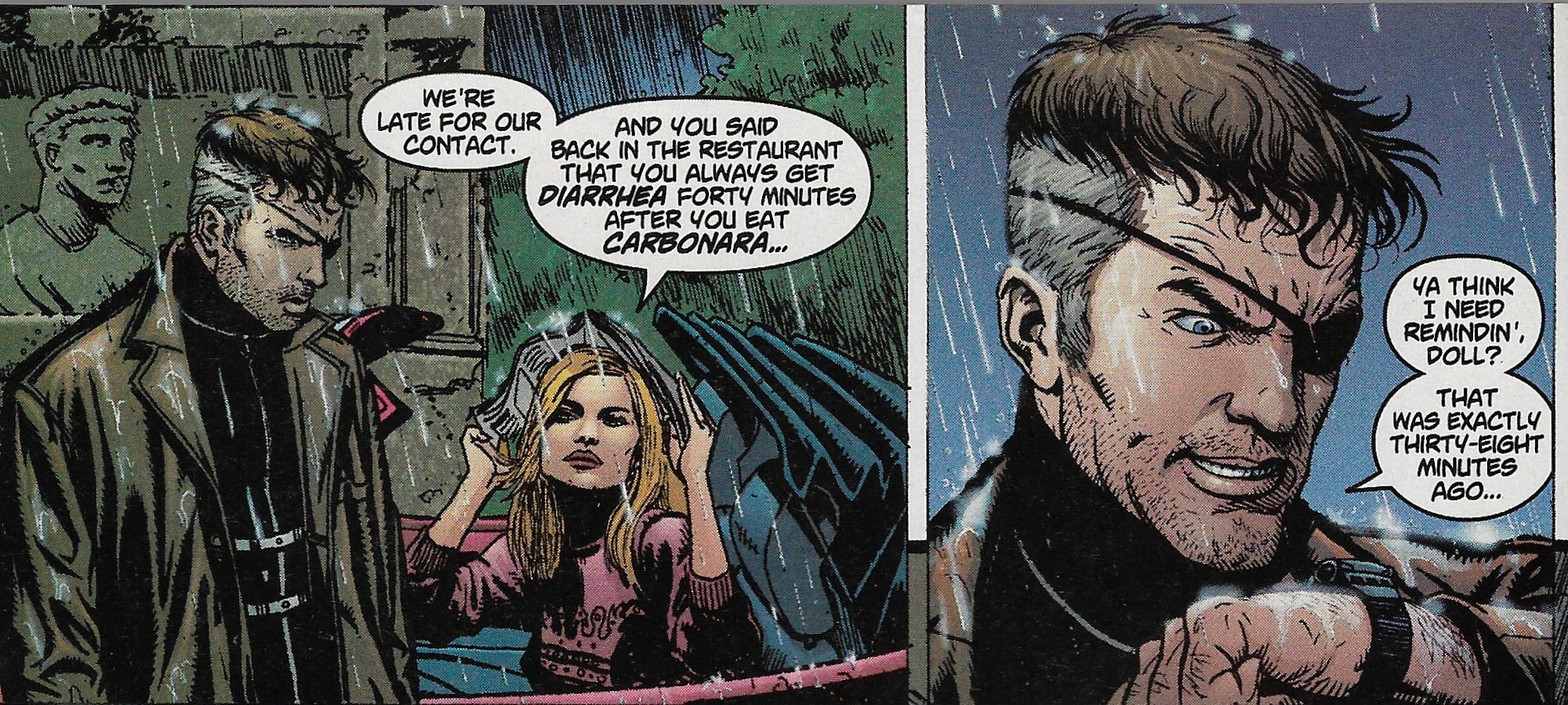This image features two consecutive panels from what appears to be a comic book, reminiscent of Marvel comics. The first panel depicts a man with an eyepatch and a woman with blonde hair standing in a heavy rainstorm. The woman, using a magazine to shield herself from the downpour, has a speech bubble above her head saying, "We're late for our contact and you said back in the restaurant that you always get diarrhea 40 minutes after you eat carbonara." The man, braving the rain without any cover, responds in the second panel. The close-up reveals his eyepatched face as he glances down at an instrument on his wrist resembling a watch. His speech bubble reads, "You think I need reminding, doll? That was exactly 38 minutes ago." The sequence humorously highlights the man's impending gastrointestinal distress, adding a unique and funny twist to their urgent situation.